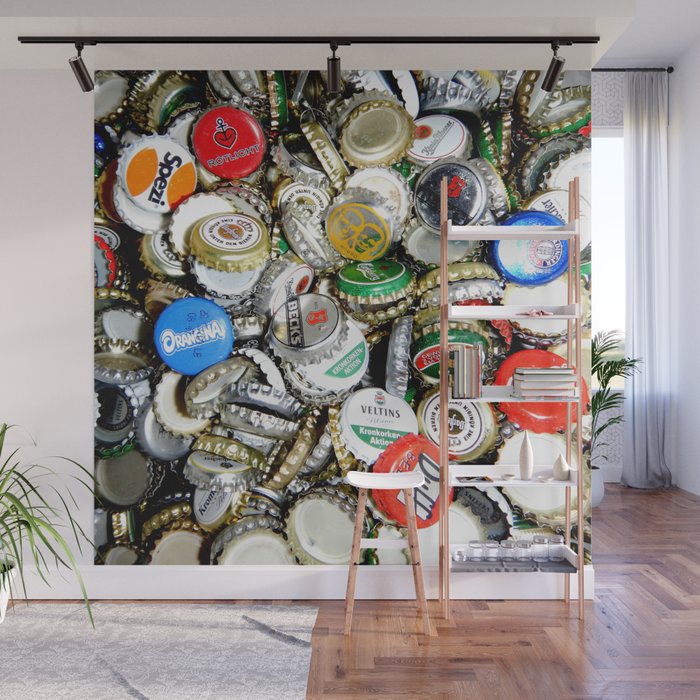The image captures a well-lit, meticulously arranged room, likely part of a private home but possibly an art gallery or stylish bar. The focal point of the photograph is an expansive mural composed entirely of scattered, unorganized bottle caps from various brands like Beck's, Orandina, Velton, Swery, and Iowa Beer. The mural, covering almost an entire white wall, creates a colorful and chaotic display emblematic of pop art. Complementing this are a high white stool, a matching white shelf filled with books and miscellaneous items, and a small potted plant on a wood floor with a cozy carpet. Above, lights are fixed to the ceiling, focusing attention on the bottle cap mural, underscoring its intended artistic statement.